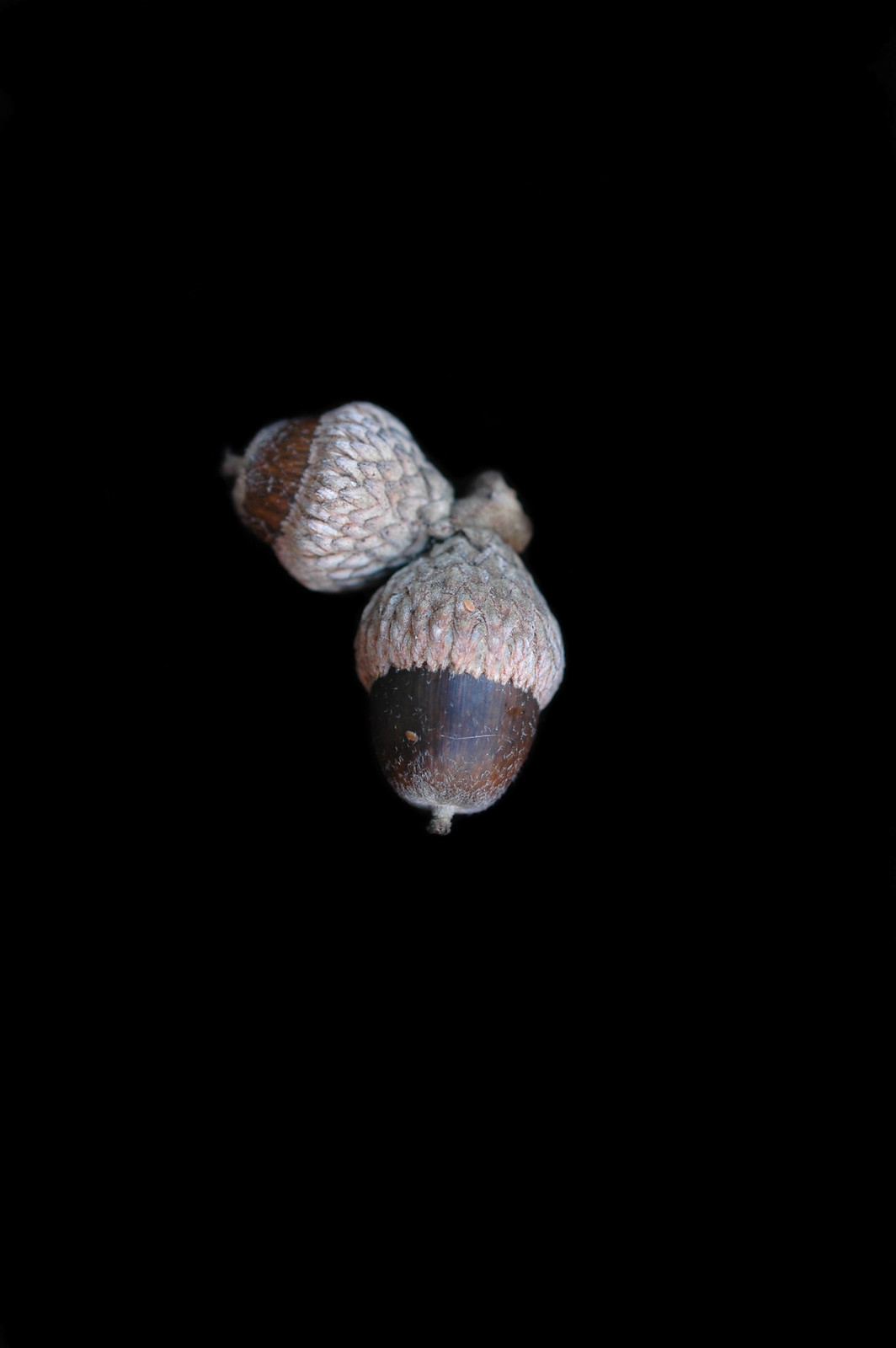The image features a close-up, detailed portrait of two acorns set against a completely black backdrop, enhancing their prominence and detail. The acorns, appearing sophisticated and meticulously arranged, are attached together at their tops by what resembles a knotted, woven string, giving the impression of a crafted or artistic approach. The acorns are adorned with textured caps that evoke the appearance of knitted winter hats in light brown and off-white hues. The larger acorn occupies the center of the image, with its smooth, dark brown body transitioning to a lighter brown towards a distinctive nib at the bottom. It is positioned such that the cap and knot are at the 12 o'clock position. In contrast, the smaller acorn is oriented at a 90-degree angle, with its cap pointing to the 3 o'clock position and its body angled towards 10 o'clock. The overall effect is a striking, minimalistic composition that highlights the acorns' unique, almost handcrafted appearance, suspended in blackness.